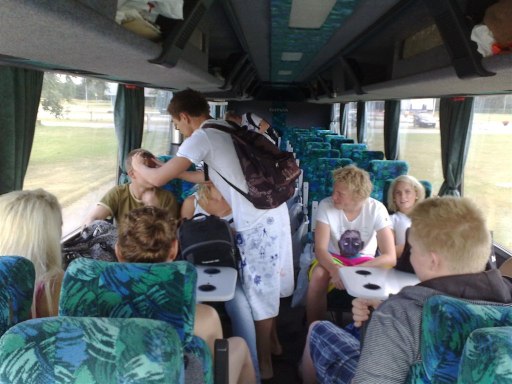In this photo, taken inside what appears to be a Greyhound or tour bus, the seats are upholstered in a tropical turquoise and green patterned felt material. The bus is filled with several young people, men and women, likely in their late teens or early twenties, all casually dressed in thin t-shirts and shorts, suggesting warm weather. The bus interior features overhead storage racks with a few items stashed away, grey curtains which are drawn back to reveal windows showing a grassy landscape with tree leaves outside.

The seating configuration suggests a close-knit group, as they are clustered together despite empty seats elsewhere. Built-in fold-out tables with cupholders are visible beside the seats. Central to the scene, a man with short scraggly hair, wearing a white ensemble with blue designs and a brown backpack, is touching the forehead of a seated gentleman, drawing the attention of the entire group. This interaction hints that they might all know each other, possibly indicating a family or friends on a tour bus expedition. The cramped space with two seats on each side of the aisle emphasizes the bus’s compact design.